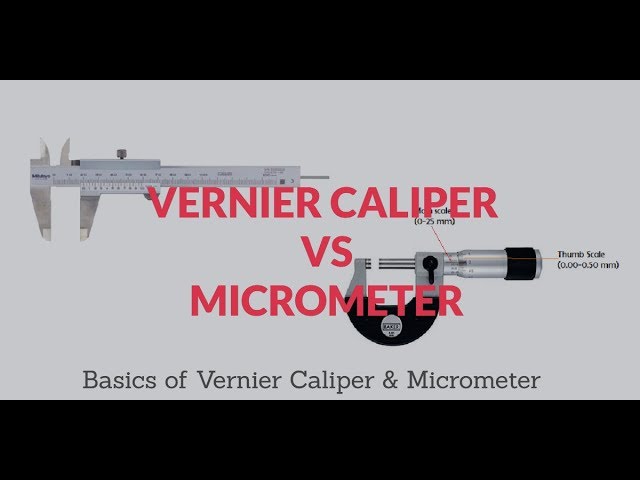The image features a cover or screenshot emphasizing a comparison between a vernier caliper and a micrometer. Framed by black bars on the top and bottom, the central area is gray with distinct elements. At the top, in bold red block letters, the title reads "Vernier Caliper Versus Micrometer." Below the title, there are visual depictions of both tools: the vernier caliper positioned on the top left and the micrometer slightly below and to the right. Both instruments are slightly opened, showcasing their measuring components. Centrally below the tools, in dark gray text, the caption states "Basics of Vernier Caliper & Micrometer." Additional textual details include a thumb scale ranging from 0.00 to 0.5 millimeters and another scale marked from 0 to 25 millimeters, emphasizing the precision usage of these tools for measuring small items. Overall, the image succinctly compares the basic functionalities of these precision measuring instruments.